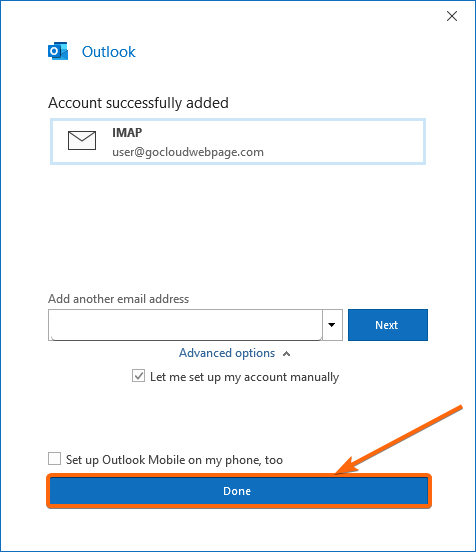The webpage displays the interface for Outlook, a popular email program, with a clean and professional color scheme of blue and white. The page is framed with a blue squared border, encapsulating a pristine white background. At the very top, "Outlook" is prominently displayed in blue letters next to a recognizable Outlook icon featuring a blue color scheme with a distinctive white "O."

Directly below the header, the message "Account Successfully Added" is presented in clear black letters. The next section features a white text box with a light blue border, prominently labeled "IMAP" in bold, uppercase letters. Beneath this label, there's an icon of an envelope which precedes the newly added email account example, formatted as user@gocloudwebpage.com. 

Following this, users are directed to "add another email address" using a provided text box. A drop-down arrow next to the text box allows for selecting other email addresses. Adjacent to this text box, a "Next" button is easily identifiable with white letters on a blue background.

Further down, advanced configuration options are available. In blue letters, "Advanced Options" is displayed alongside a black upward arrow. Below, the option to "let me set up my account manually" appears in black letters, marked by a checkbox indicating that this preference has been selected.

Additionally, there's an option to "set up Outlook Mobile on my phone too," accompanied by an unselected checkbox.

At the very bottom of the page, the word "Done" is visible in white letters on a blue background. This element is accentuated with a thick red border and an attention-grabbing red arrow pointing directly at it, guiding users towards the next step in the setup process.